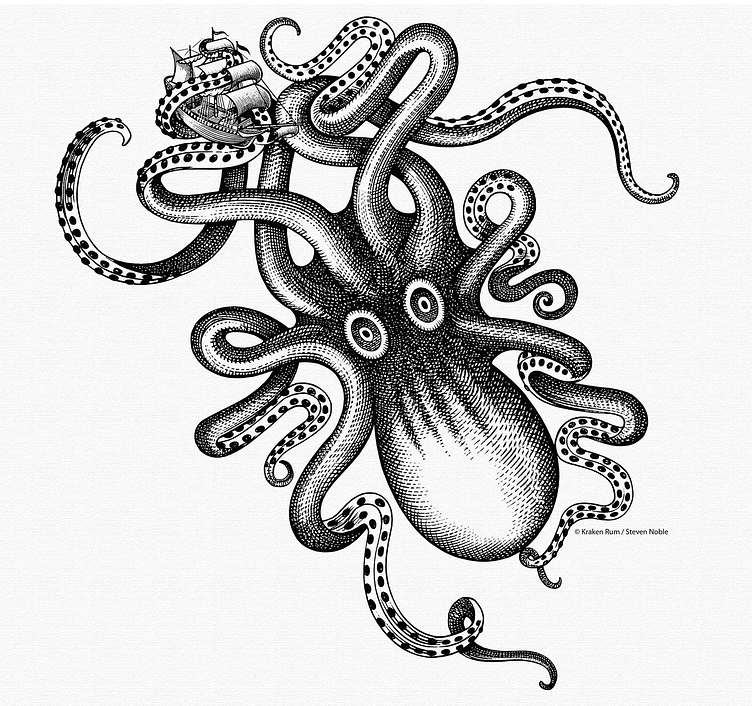This black-and-white artwork, created by Stephen Noble for Kraken Rum, depicts a colossal Kraken or giant squid dominating the scene. The giant squid's bulbous head, which features two large, staring oval eyes, points downwards to the right. It is surrounded by eight sinuous tentacles, shaded in black and white, some of which spiral intricately around each other. One of these powerful appendages notably wraps tightly around a small sailboat located at the upper left of the image, emphasizing the immense scale of the Kraken. The sailboat, equipped with white sails and devoid of crew, appears minuscule in comparison to the massive creature. The detailed illustration also includes a copyright notice at the bottom, reading "KrakenRum/Stephen Noble."